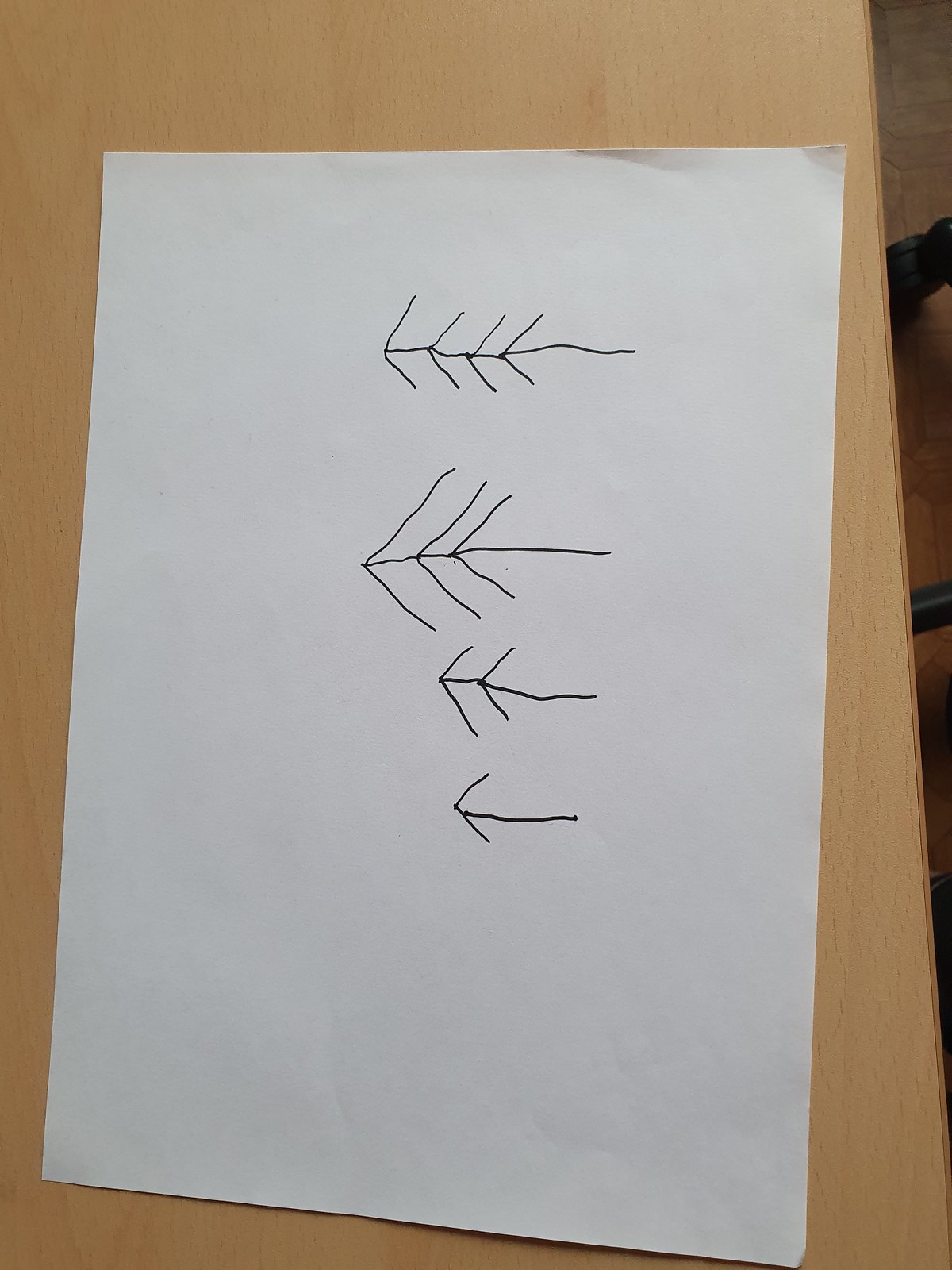The image features a light-colored wooden table or desk, partially revealing a tile-like floor and a few indistinguishable elements that might be parts of a chair. Dominating the table surface is a rectangular piece of white paper. The paper is marked with lines in either a thin black marker or a very dark pencil. Positioned from slightly below the top to the middle of the paper are four arrows, all pointing left. Each arrow's head varies; the topmost arrow has four pointed sections behind the tip, the next arrow has three, followed by one with two sections, and the last has only one pointed section. The purpose or context of these arrows is unclear.